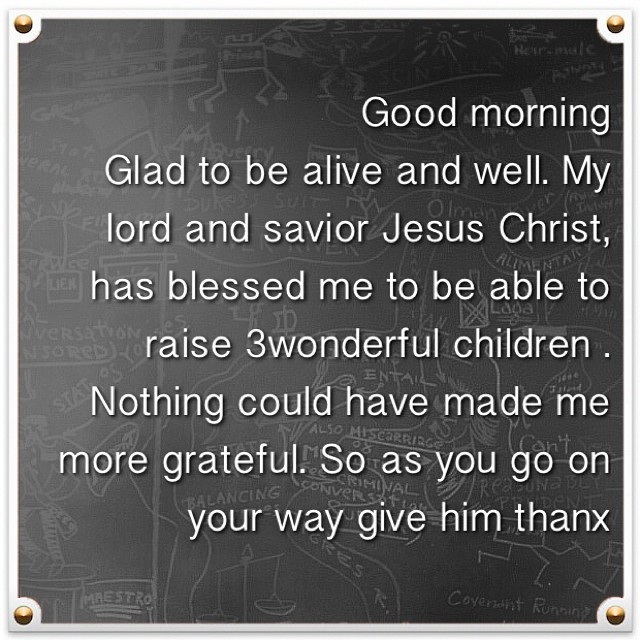The image features a Christian-themed message displayed within a framed write-up. The frame has a white border with each corner adorned by a golden-colored pin. The background is gray and adorned with faint, light gray scribbles of drawings and texts, resembling a chalkboard. The central message, written in white text, reads: "Good morning, glad to be alive and well. My Lord and Savior Jesus Christ has blessed me to be able to raise three wonderful children. Nothing could have made me more grateful. So as you go on your way, give him thanks." Notably, the word "thanks" is spelled as "T-H-A-N-X". The phrase "three wonderful children" is written without a space between "three" and "wonderful", and there is a space before the period following the word "children". The overall aesthetic resembles that of a Christian social media meme, with the design elements giving it a historical monument-like appearance.